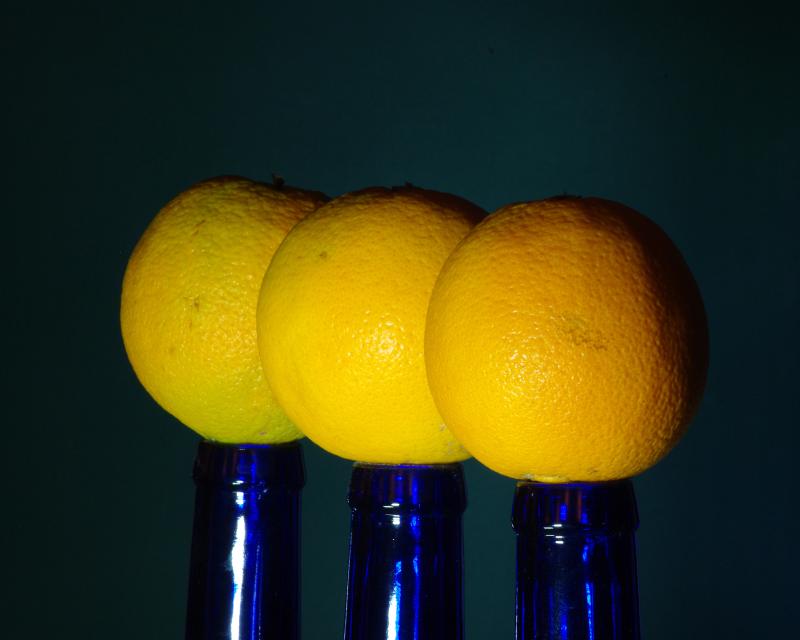In this photograph, we see a dark background that fades from charcoal gray to black, highlighting the central subjects. Three bright oranges, each displaying tiny blemishes, rest individually on the tops of blue glass bottles. Only the bottle necks are visible, suggesting they might be beer or water bottles with low necks. The oranges, ripe and full, cast a shadow that stretches from the top right corner across them, indicating a light source coming from the bottom right. The first orange on the left has a hint of green, showing it might not be fully ripe. Light reflections on the blue glass add a subtle gleam, emphasizing the bottles' smooth surface. The positioning and lighting make the oranges and bottles the clear focus of this minimalist, yet intriguing image.